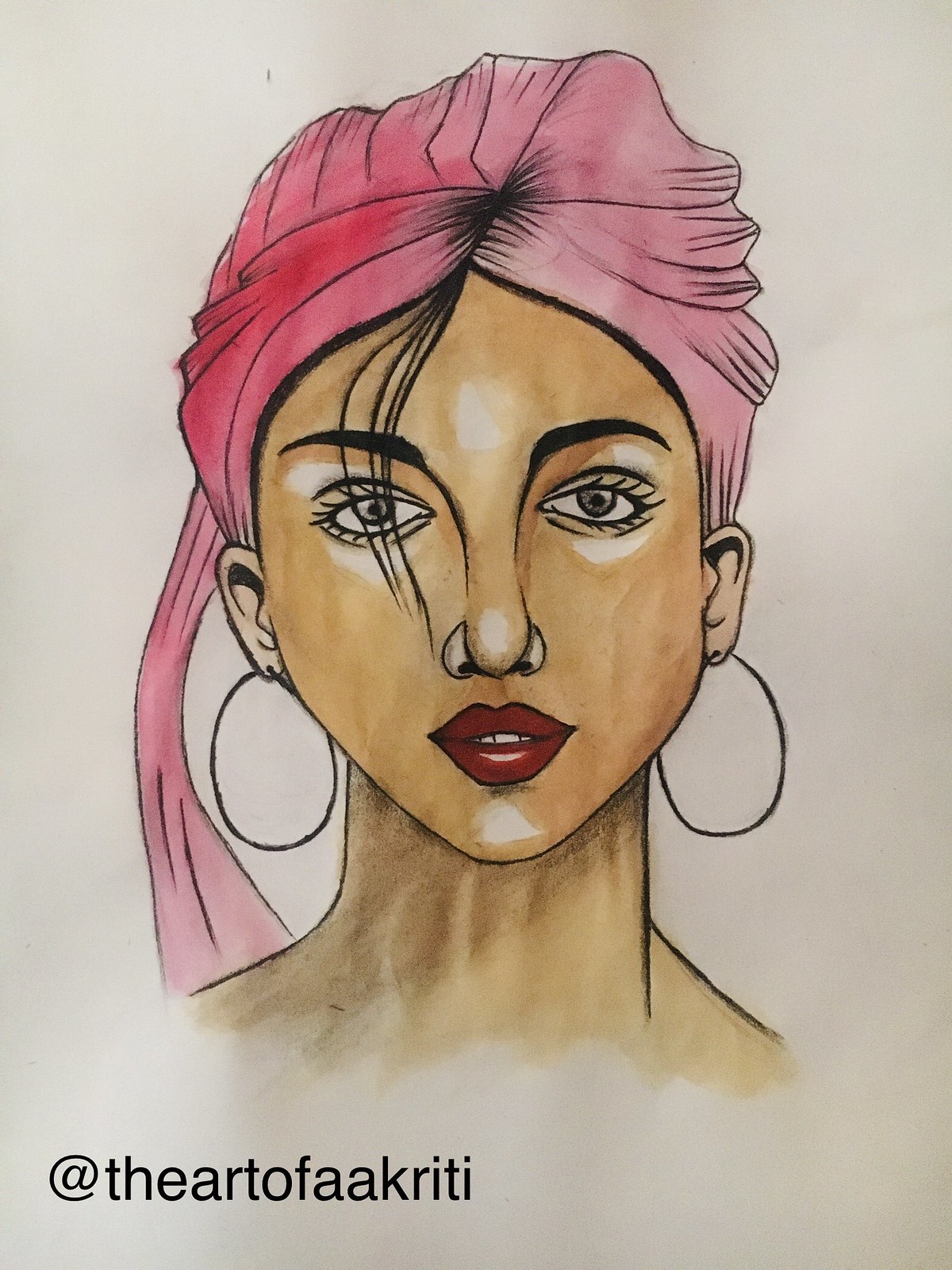In the image, there is a white piece of paper displaying a colorful drawing. The medium used appears to be either paint or colored pencils. At the bottom of the image, the text "@TheArtOfAakriti" is written in black. The drawing features a light-skinned woman wearing a pink headwrap, which is darker on the left side and lighter with black outlines on the right. Her black bangs partially cover her right eye, which is on the viewer's left side. The woman's eyes are gray, and she has black, arched eyebrows framing her oval-shaped eyes. She is adorned with red lipstick, and her slightly open mouth reveals her teeth. She is also wearing black hoop earrings. The drawing shows her neck, but does not extend further down.